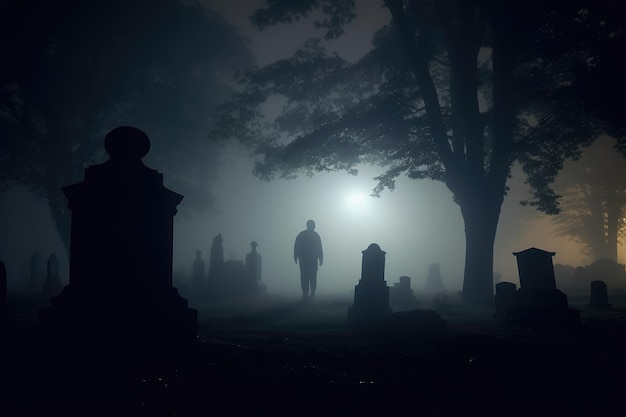In this eerie, monochromatic depiction, a silhouette of a solitary figure, appearing to be a man, is seen walking through a graveyard shrouded in dense fog. The scene is lit by a dull, haunting light source, possibly a full moon, casting an otherworldly glow over the entire landscape. The graveyard is dotted with various tombstones and crypts of diverse shapes and designs, their silhouettes adding to the macabre atmosphere. Large, shadowy trees frame the setting on the right and in the background, their branches like skeletal fingers reaching out through the mist. The central figure's indistinguishable direction and the pervasive mist create an unsettling, ethereal ambiance, making it hard to discern whether this image is a photograph or a masterfully crafted piece of fantasy horror art.